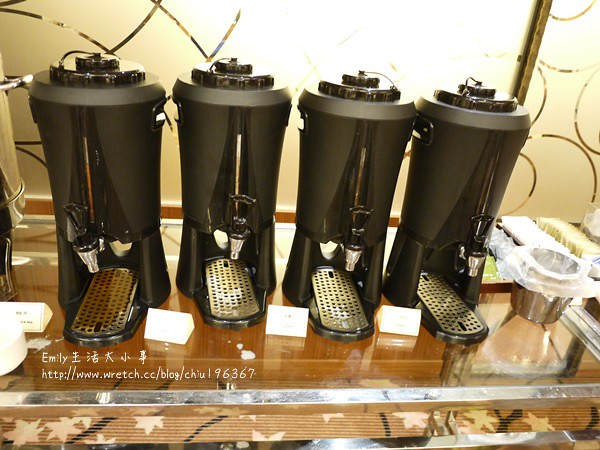This detailed photograph captures four large black cylindrical beverage dispensers, each equipped with a silver spout and a black handle located above a steel metal drip grate with multiple holes. The canisters are neatly arranged on a glass countertop framed with silver steel. The background features a tan, blank painted wall illuminated by a white light, while the base of the room reveals a brown backdrop. On the bottom left of the image, the text "Emily" is visible in white accompanied by Chinese characters and a URL linking to a blog page. In front of each dispenser, small tags and a metal cup lined with plastic add to the organized presentation. The scene is subtly decorated with a pattern of brown stripes and faint white stars across the front of the display case, contributing to the overall aesthetic.